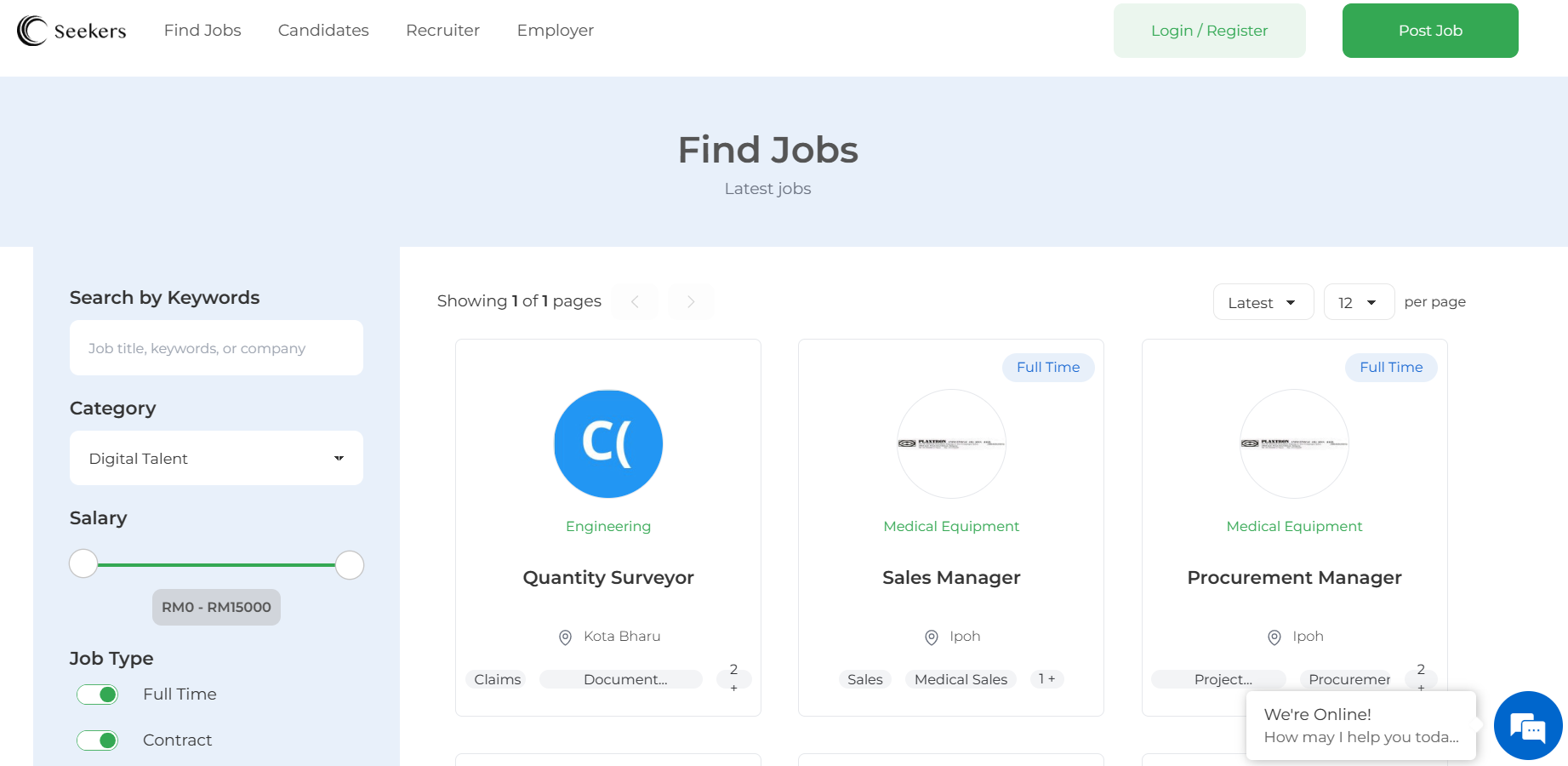The image depicts a screenshot of the Seekers website interface. Dominating the top of the page is the Seekers logo, characterized by a stylized black wave swirling around the letter "C" adjacent to the word "Seekers" written in black letters. Just to the right of the logo, the tagline "Find Jobs" appears in gray text. Other menu options such as "Candidates," "Recruiter," and "Employer" also feature the same gray typography, providing easy navigation across the site.

At the very top of the page, there are additional navigation buttons labeled "Log In / Register" and a prominent green button labeled "Post Job."

The main section of the webpage showcases job listings under the heading "Find Jobs" and a subheading "Latest Jobs." The first listing is for an "Engineering Quantity Surveyor," followed by a "Sales Manager" position for medical equipment, and concluding with a "Medical Equipment Procurement Manager" role on the far right. Notably, the "Sales Manager" and "Procurement Manager" listings are marked with an oval label in the top right corner of their respective rectangles, indicating that these positions are "Full Time."

At the bottom of the webpage, a customer support chat interface is visible, represented by speech bubbles. The chat prompt reads, "We're online. How may I help you today?" followed by an ellipsis, suggesting that the conversation is ongoing or awaiting user input.